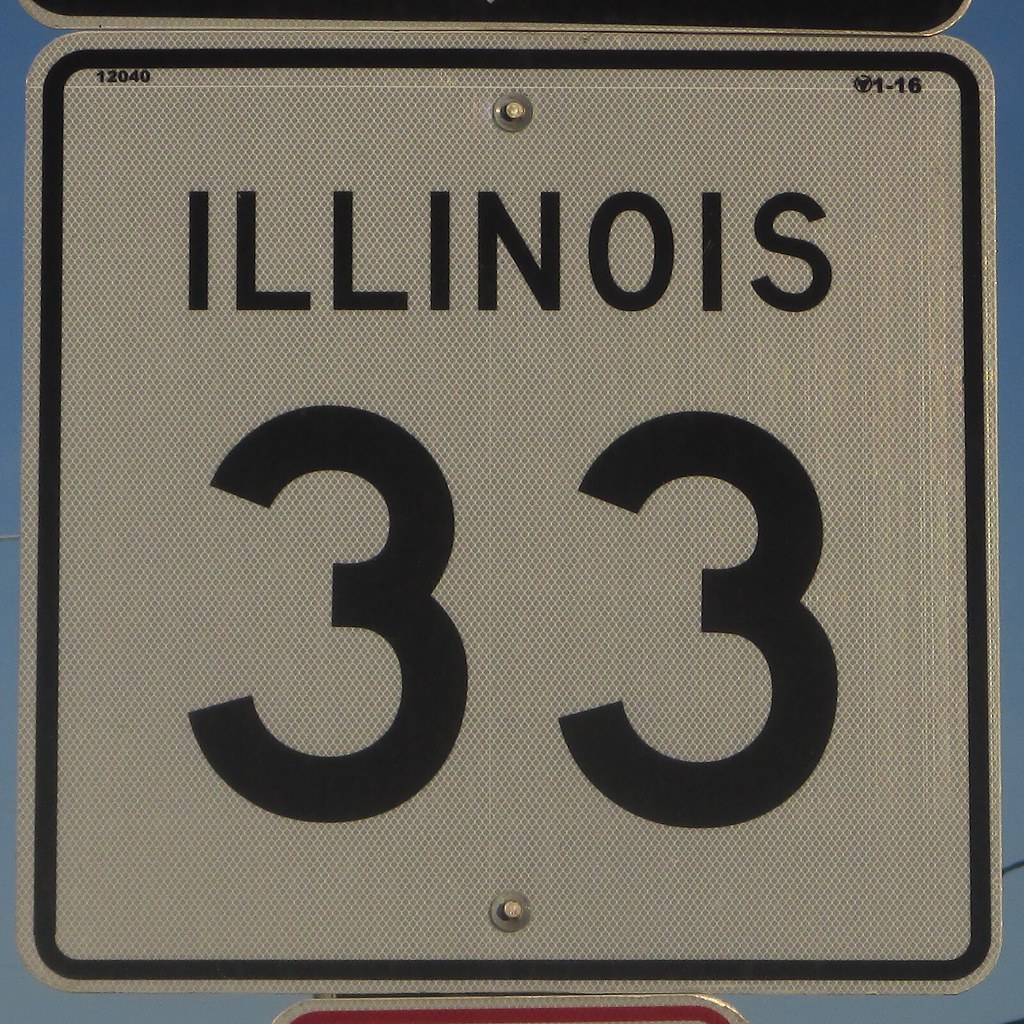The image showcases a roadside sign prominently featuring the state of Illinois. The square sign is bordered with a black outline, adding a distinct frame to its white background. At the center of the sign is the large number "33," which is printed in bold, big black font. Above the number, "Illinois" is displayed in a medium-sized black font relative to the size of the sign. In the top left corner, the number "12040" is printed in very small, precise characters. The top right corner also contains small print, though it is somewhat difficult to decipher; it appears to include a small icon followed by the digits "1-16." 

The backdrop of the sign is a clear, medium blue sky, creating a crisp and clean contrast with the black and white sign. Below the Illinois sign, a hint of another sign is visible, characterized by red and white coloring. Additionally, there is another sign at the top, similar in color scheme to the Illinois sign. The overall image is sharp and provides a clear view of the landmark sign.